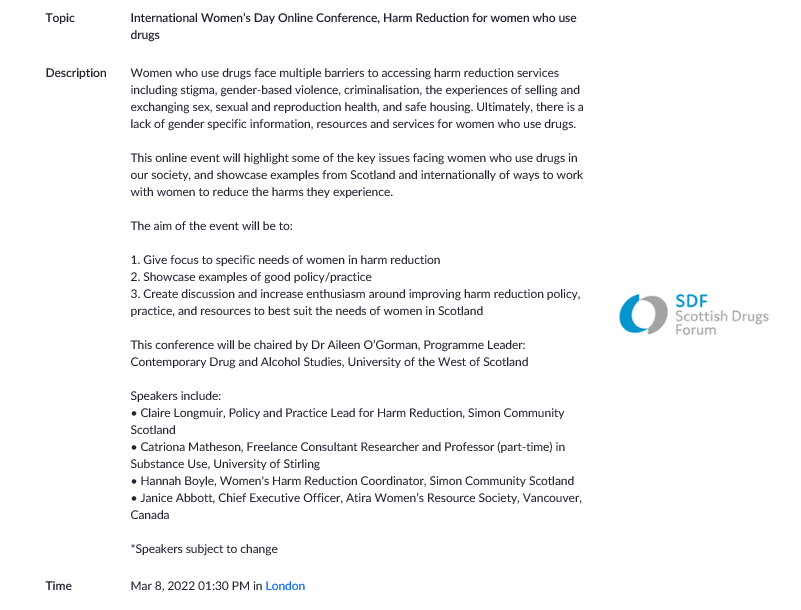**Caption:** 

This image contains detailed information about an upcoming online conference titled "International Women's Day Online Conference: Harm Reduction for Women Who Use Drugs." The event focuses on the multiple barriers women face in accessing harm reduction services, such as stigma, gender-based violence, criminalization, and experiences related to sex work, sexual and reproductive health, and safe housing. There is a noted lack of gender-specific information, resources, and services for women who use drugs.

The conference aims to:
1. Address the specific needs of women in harm reduction.
2. Showcase examples of effective policy and practice.
3. Generate discussion and enthusiasm around improving harm reduction policies, practices, and resources tailored for women, particularly in Scotland.

Dr. Eileen O'Gorman, Program Leader of Contemporary Drug and Alcohol Studies at the University of the West of Scotland, will chair the event. Featured speakers include Claire Longmuir of Simon Community Scotland, Ketch Rhiona Matheson, a freelance consultant and part-time substance use professor at the University of Stirling, Hannah Boyle, Women's Harm Reduction Coordinator at Simon Community Scotland, and Janice Abbott, CEO of ATIRA Women's Resource Society in Vancouver, Canada. Note that speaker participation is subject to change.

The conference is scheduled for March 8, 2022, at 1:30 p.m. London time. The image also features the logo of the Scottish Drugs Forum (SDF).